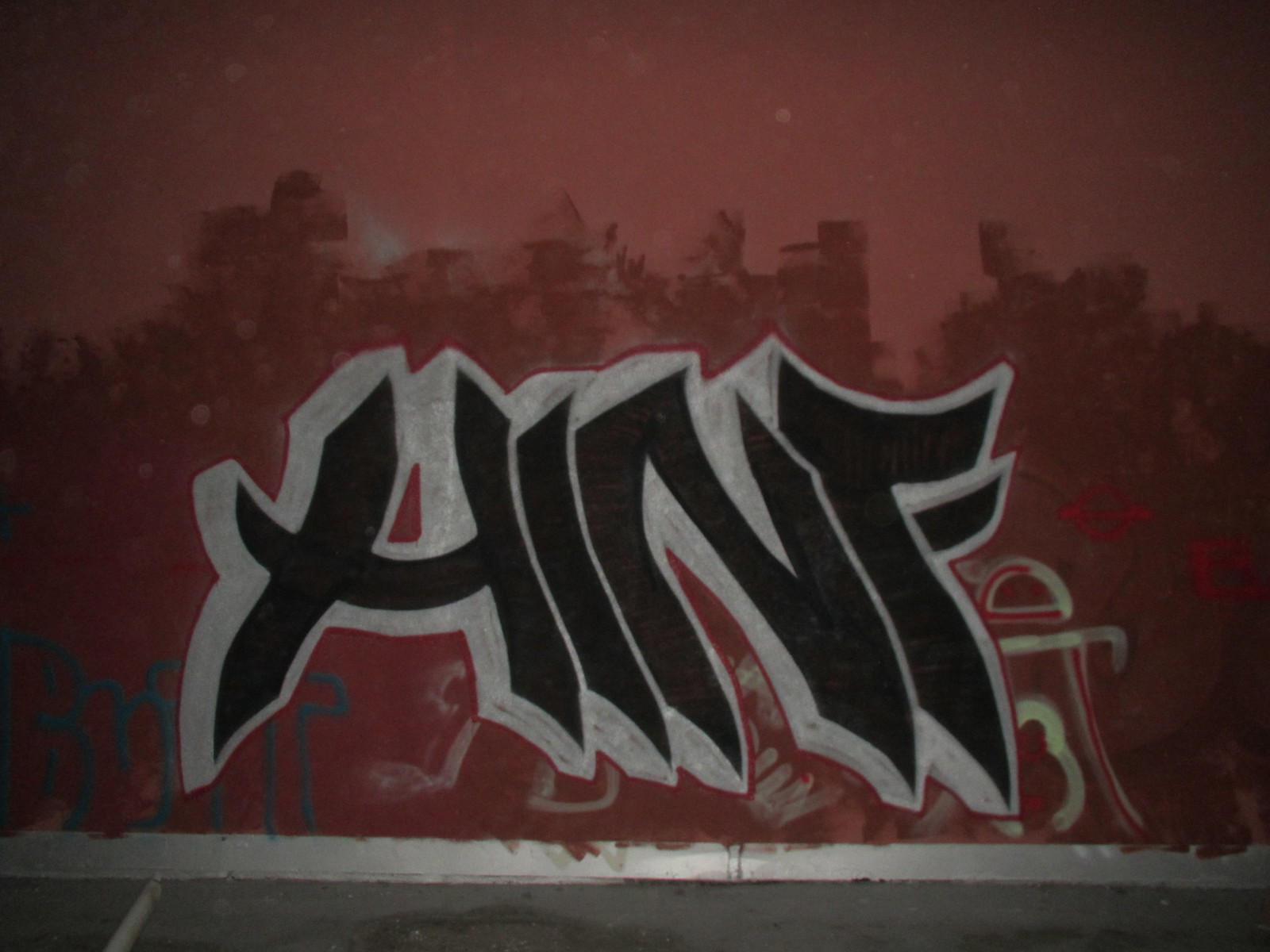The image captures an outdoor nighttime scene, likely in a parking lot. At the bottom, an asphalt road with a white painted stripe meets a prominently featured red wall. This wall, originally lighter red, has been overlaid with rough strokes of darker red paint. At the center of the wall, large, curvy graffiti letters in black and white spell out "A-I-N-F", outlined in white. Surrounding the letters, there are whimsical green and blue doodles. The overall color palette includes gray, white, blue, black, maroon, pink, and varying shades of red. The graffiti commands the focus of the image, framed by the contrasting textures and colors of the paved ground and painted wall.